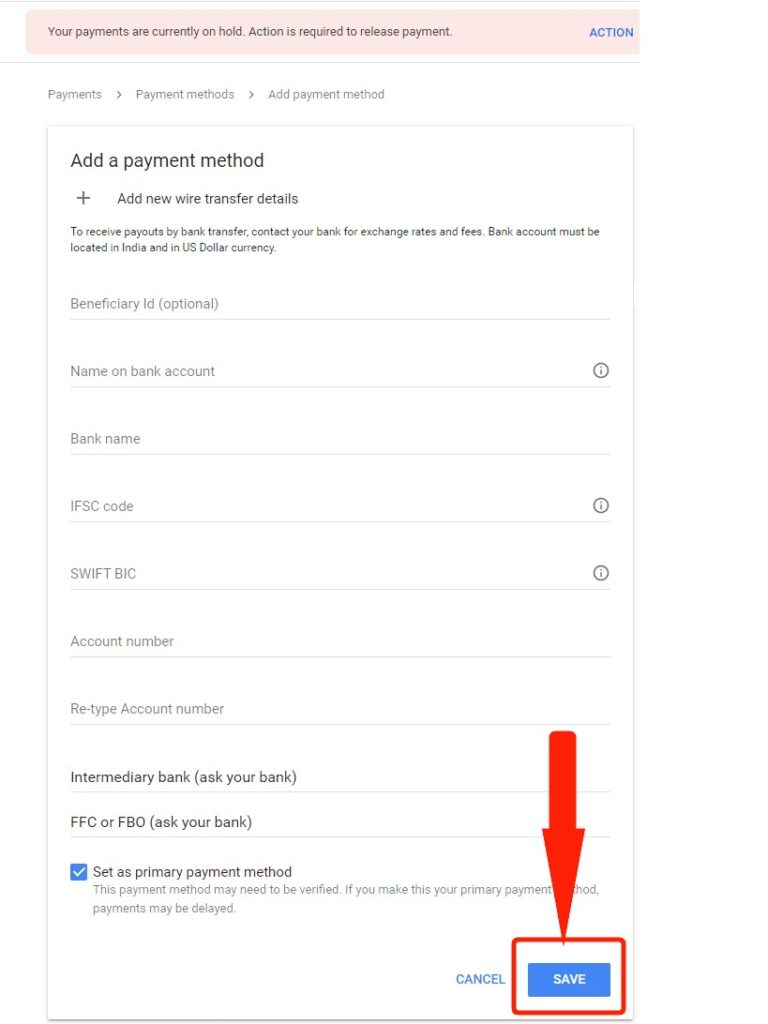This image depicts a webpage for adding a payment method, prominently featuring a disclaimer at the top in a pink box that states: "Your payments are currently on hold. Actions required to release payment." To the right of this disclaimer is a blue action button labeled "Payment Methods," which navigates users to the payment methods page, where they can add a new payment method.

The page currently shows the section to add a new payment method. At the top of this section, in darker black text, it says "Add a Payment Method," with a plus sign indicating the addition of new wire transfer details. It includes a detailed description of how to proceed, mentioning: "See payouts by bank transfer. Contact your bank for exchange rates and fees."

Below this, there is a form where users can enter various details:
- Beneficiary Name
- Bank Account
- Bank Name
- IFSC Code or SWIFT/BIC Code
- Account Number
- Confirm Account Number

The fields above are primarily grayed out, implying they may not be editable at the moment. 

Further down, there is a field for adding an Intermediary Bank, with advice to "Ask your bank about this." This field is slightly darker than the others and labeled "FFC or FBO" with a note to ask the bank for the correct information.

Additionally, there is a checked checkbox labeled "Set as primary payment method" with a note that says: "Payment method may need to be verified to make it your primary payment method. Payments may be delayed."

At the bottom right corner of the page, two buttons are available:
- A blue "Cancel" button
- A white "Save" button with a blue border

There is also a massive thick red arrow pointing down towards the "Save" button, emphasizing its importance.